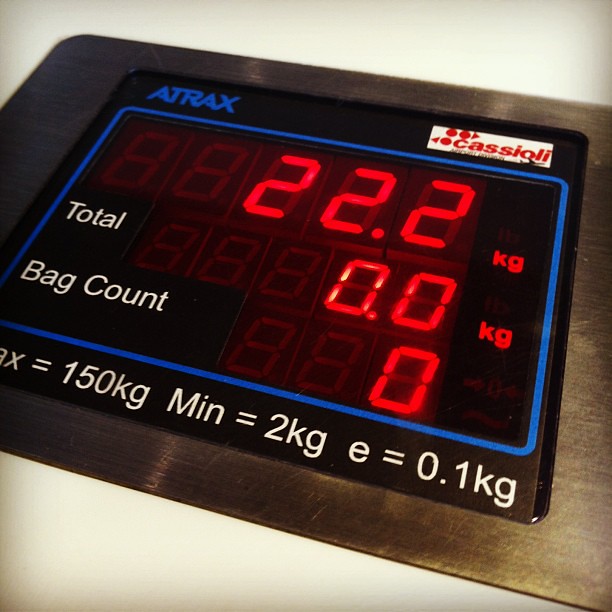The image displays a detailed view of a digital scale. The scale features a metallic gray outer casing with a central display area set against a white background. On the upper left of the display, the brand name "ATRAX" is prominently featured in blue text. On the upper right, within a white square, the logo "CAS" is clearly visible in red lettering. The digital readout itself is housed in a black inset with bright red electronic numbers. The display shows three lines of text: the top line reads "22.2 kilograms," the next line reads "total 0.0 kilograms," indicating the total weight, and the final line shows "bag count zero," all in red. Detailed specifications are printed in white text along the bottom of the scale, stating "MAX equals 150 kilograms, MIN equals 2 kilograms, E equals 0.1 kilogram." This scale appears to be designed for weighing bags, perhaps for shipping or packaging purposes.